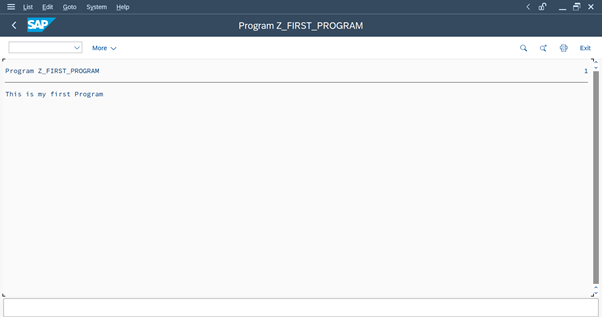This screenshot captures a webpage layout from an SAP system interface. At the top left, the SAP logo is prominently displayed in white text against a blue background. The top header, which spans the full width of the page, is black and includes text elements such as "Small Images" and "Help System," though some text remains unreadable due to its small size. Centrally located within the header is the title "Program Z_first_program." 

On the top right corner of the header, there are several small, indistinct icons. Directly below the header, a search bar is visible, featuring a down-arrow indicator and the word "More" with another down-arrow icon beside it. To the right of the search bar, a set of blue icons is present. 

Beneath the search bar, the title "Program Z_first_program" is displayed again, underlined for emphasis. Following the title to the right is a small number "1," possibly signifying an index or list number. Below the underline, the text "This is my first program" appears, formatted in a bluish-purple hue. Adjacent to this text, a vertical gray scrollbar runs down the right side of the page, indicating additional content can be viewed by scrolling. 

Finally, at the bottom, where the webpage content ends, a plain white bar spans the width of the page, serving as a footer or boundary.